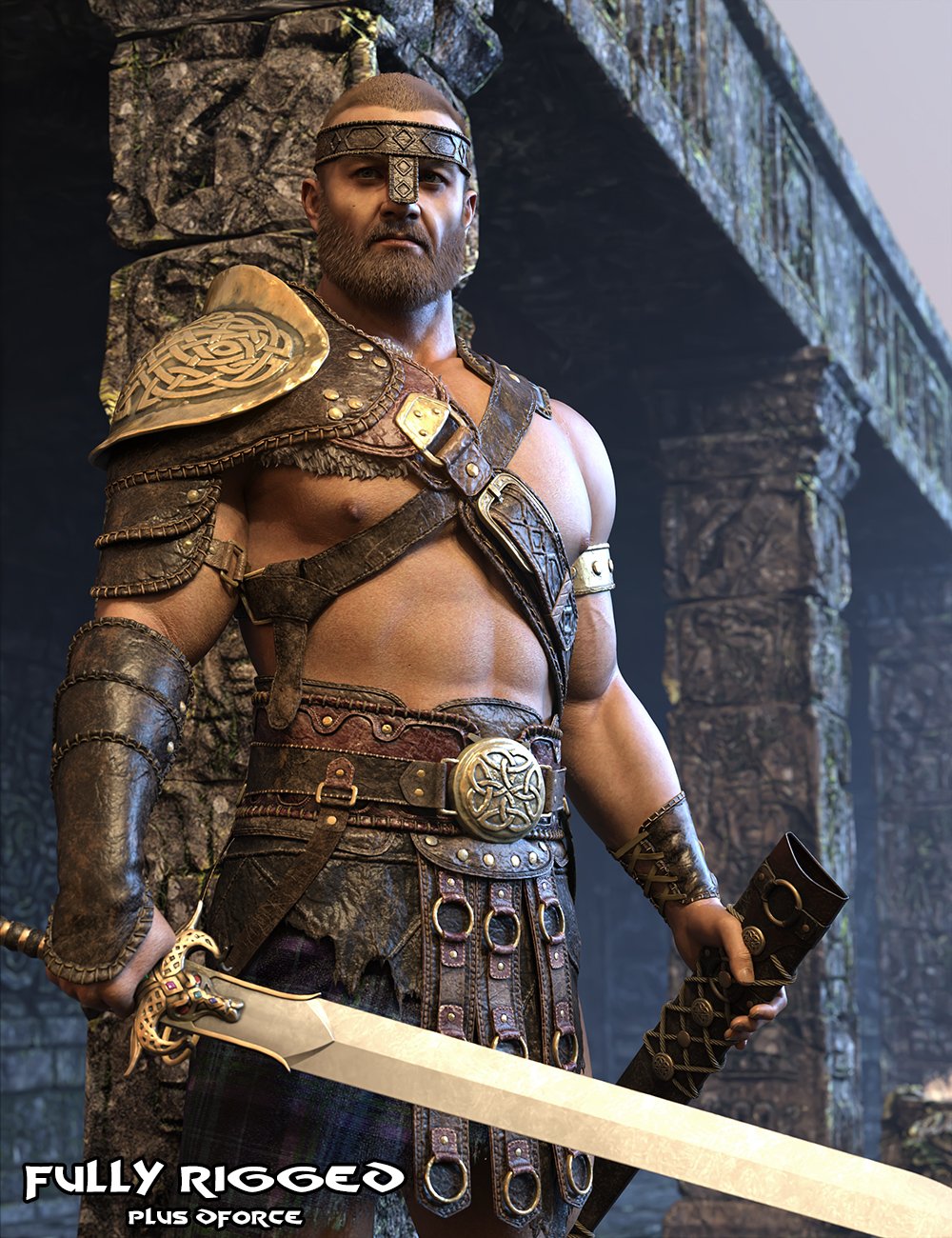This detailed 3D rendering depicts a muscular man dressed in gladiator-like armor. He is bare-chested with brown leather straps crisscrossing his torso and a thick brown beard. Short brown hair tops his head, and a brown strap around his forehead extends over his nose. His left shoulder is adorned with a gold-colored piece of armor accented with brown, yellow, and orange rivets. His left arm hangs down, showcasing a heavy leather forearm guard extending from elbow to wrist. Gripping a large, downward-facing sword with a yellow blade in his left hand, he holds its ornate sheath in his right. A Celtic-inspired bronze medallion sits at his navel, and he wears a kilt-like skirt with leather details. The background features ancient stone structures reminiscent of a dark granite Colosseum. At the bottom left, text in white capital letters with a black border reads "FULLY RIGGED PLUS FORCE."